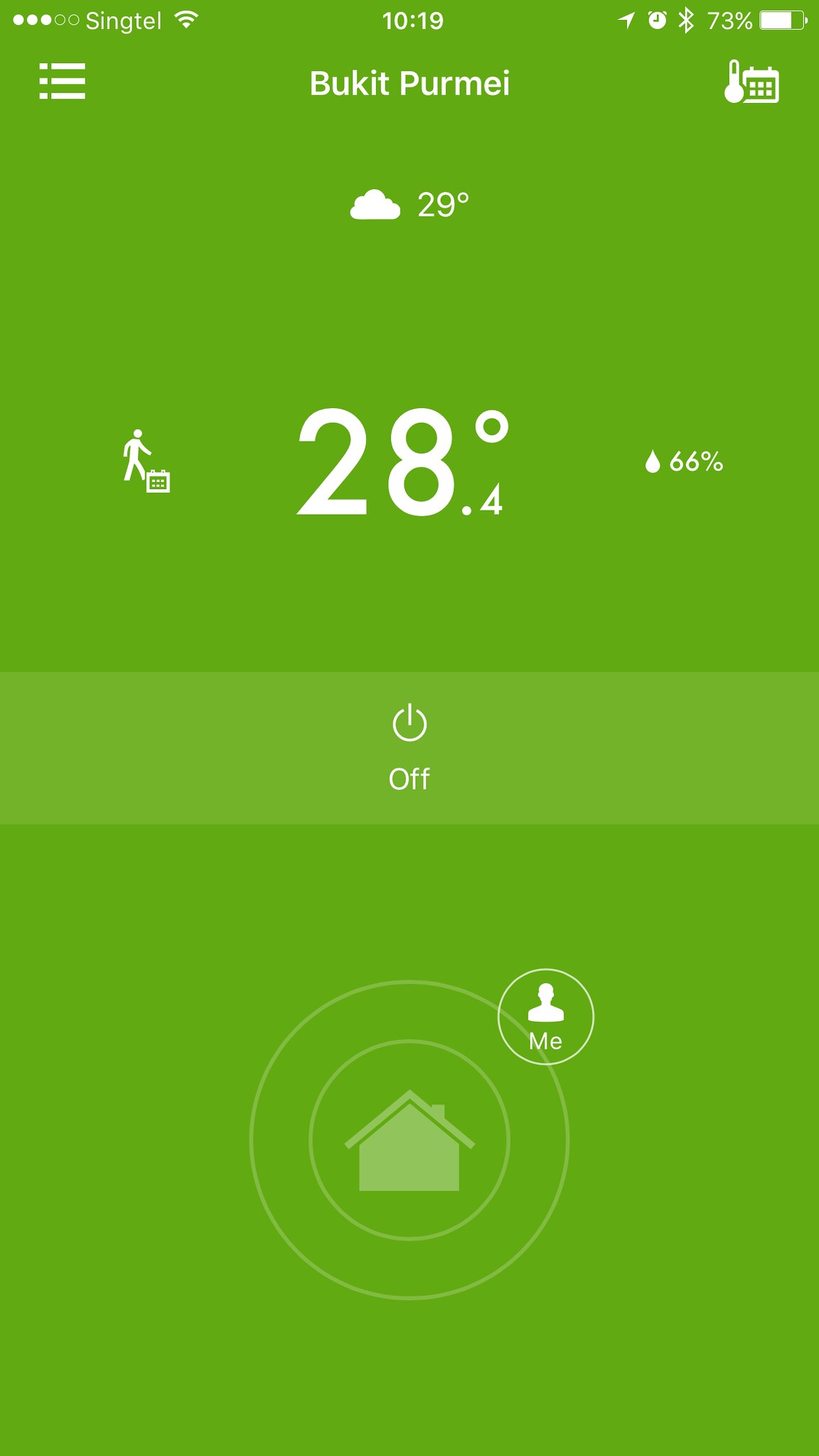In the image, which appears to be a screenshot taken from an iPhone, several interface elements and details are visible. The top of the screen displays typical iPhone icons: the battery percentage is at 73%, with the current time showing as 10:19 AM. Additionally, the Bluetooth and location icons are visible alongside the Singtel network name, indicating the phone service provider, with Wi-Fi and signal bars displayed.

On the upper left corner, there are three horizontal lines suggesting a menu icon, and beneath this is the text "Book it for me," likely in another language. Below this, the temperature is displayed as 29°C, accompanied by a cloud icon.

Further down, there's an illustration of a stick figure walking to the right with a calendar icon beneath it showing "28.4°C" and "66%" next to raindrop symbols, suggesting a 66% chance of rain. In the middle of the screen, an off button is prominently featured.

At the bottom, there is a house icon with two circles around it, next to which it says "Me" accompanied by a silhouette of a person representing a profile icon.

The background color of the interface is green, tying all these elements together.